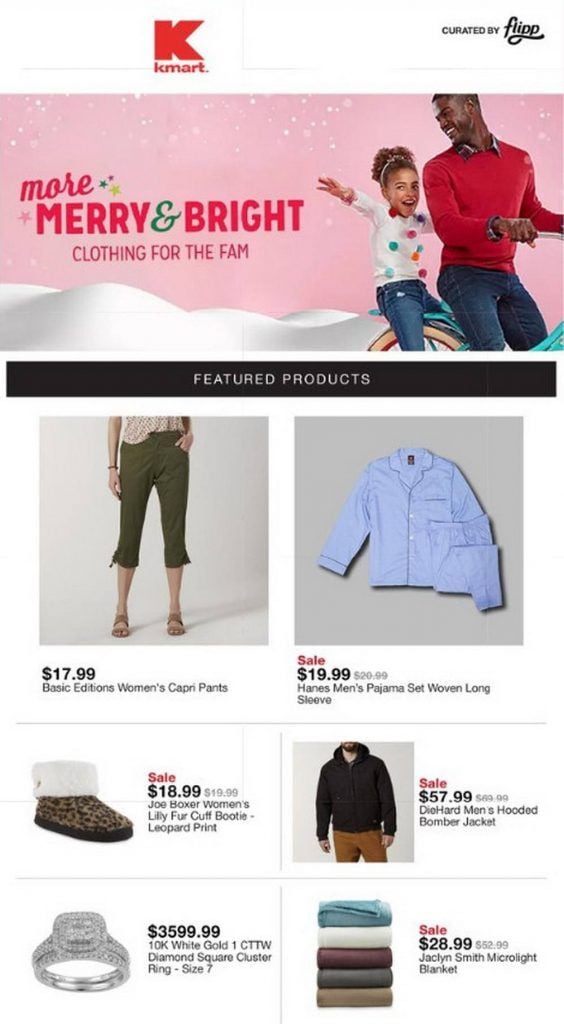This image is a screenshot taken from the Kmart shopping site. The top section of the image features a clean white background. In the upper right-hand corner, it's marked with the phrase “Curated by Flip,” written in elegant script. On the upper left center, Kmart's logo is clearly displayed.

Dominating the center of the image is a large festive photograph set against a pink background adorned with little snowflakes. The text "More Merry and Bright Clothing for the Fam" is prominently displayed. The photo showcases a joyful scene with a dark-skinned young girl and a dark-skinned male riding a bicycle, both dressed in jeans. The male is wearing a red sweater, while the girl sports a white sweater with polka dots, her arms outstretched in delight as both smile brightly.

Beneath the photo, a black stripe announces "Featured Products." The next row is split into two images: on the left, there are olive-colored capri pants labeled "Basic Editions Women's Capri Pants - $17.99." Only the woman’s legs and sandals are visible. To the right is a light blue Hanes Men's Pajama Set, meticulously folded and marked "Woven Long Sleeve Pajama Set - Sale $17.99" in red.

The following row displays more products. On the left side is an image of a slipper with the label "Sale $18.99 Joe Boxer Women's Lily Fur Cuff Booty Leopard Print." On the right side is a picture of a hoodie and brown pants with the text "Sale $57.99 DieHard Men's Hooded Bomber Jacket."

Finally, the bottom row features two more items: on the left is a diamond ring, and on the right is a neatly stacked pile of blankets, completing the array of holiday-inspired offerings.